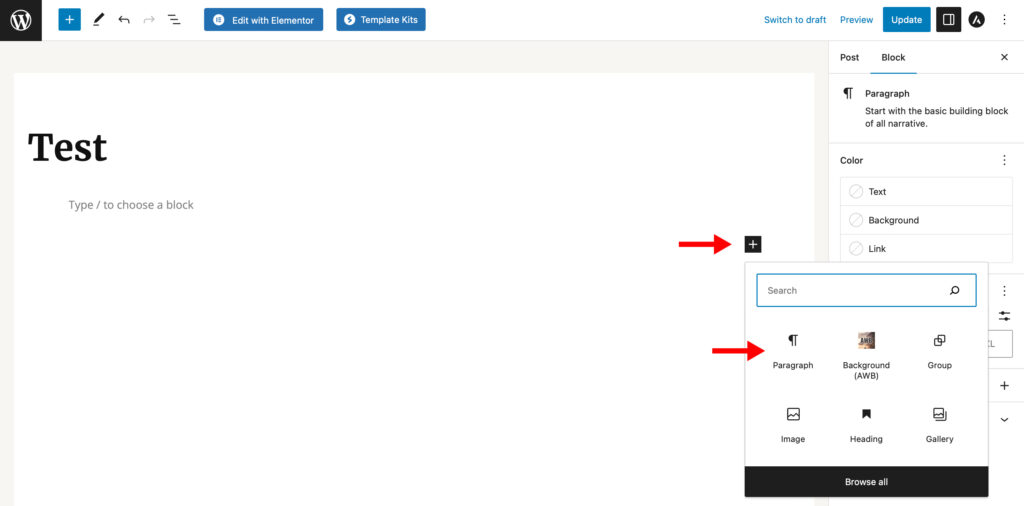**Detailed Caption:**

The image features a detailed interface of a WordPress editing screen with a clean white background. In the top left corner, there is a distinctive black icon on a circular white background, showcasing a bold, capitalized letter "W" in white writing. Adjacent to this icon is a blue button with a white plus symbol. Following this, there is a pin button, succeeded by an arrow icon that indicates navigation options pointing both directions. Next, three horizontal lines can be seen, followed by a button labeled "Left with Elementor," and another button labeled "Template Kits."

Moving further to the right, there are labeled buttons reading "Switch to Draft," "Preview," and "Update." Beyond these, there are two additional unrecognized icons. Under this entire section, the header prominently displays the word "Test" in large black font towards the left. 

On the right side of the screen, the words "Post" or "Block" are visible, and beneath that, a section labeled "Paragraph" with sub-sections for "Color." This color section is divided into three bubbles labeled "Text," "Background," and "Link." Below this is a search bar, above which there's a black plus button marked with a red arrow pointing towards it.

Additionally, another red arrow points to the word "Paragraph" located under the search bar. In the central part of the interface, there are six labeled components arranged in two rows. The first row includes: "Paragraph," "Background," and "Group." The second row consists of: "Image," "Heading," and "Gallery." At the bottom, there is a prominent black button labeled "Browse All."